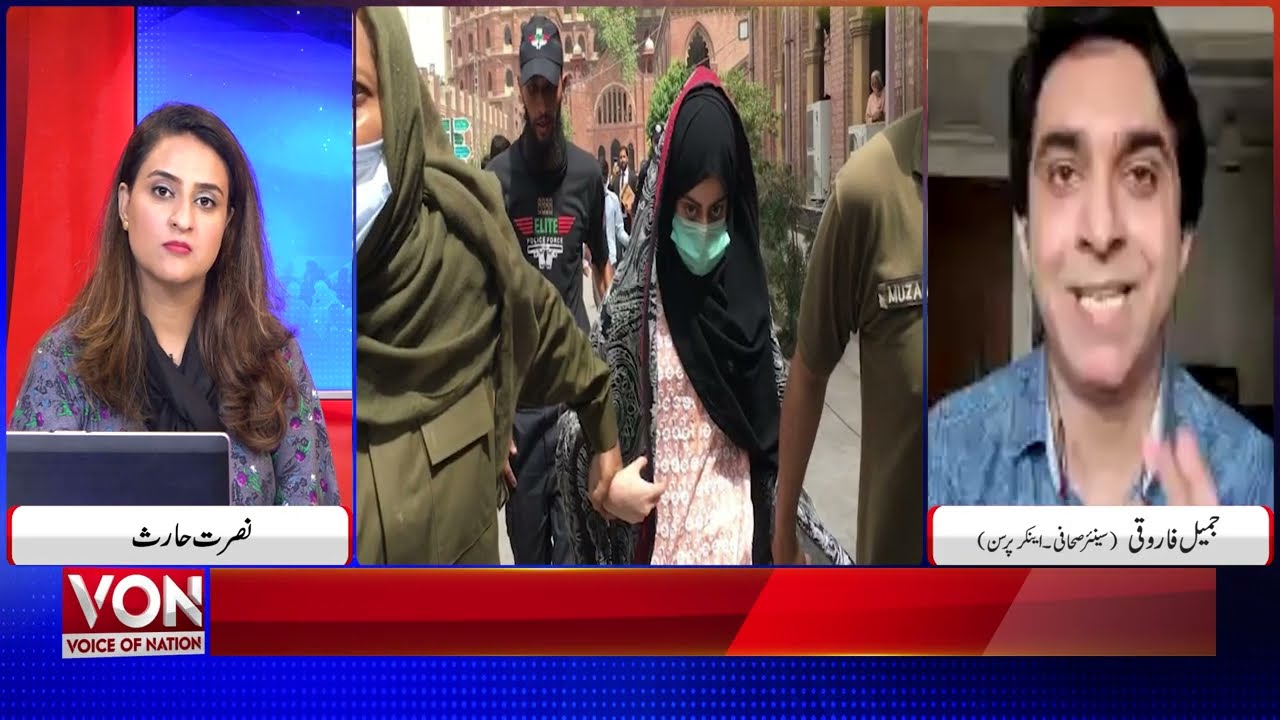The screenshot depicts a news broadcast segmented into three distinct panels. On the left, a female news anchor with olive skin, long dark hair featuring reddish-blond highlights, and a dark floral shirt paired with a scarf, sits behind a computer on a blue and red background. The text at the bottom of her panel reads "Vaughn, Voice of the Nation." To the right, a male interviewee with dark black hair and a jean jacket appears mid-conversation, facing the camera with an animated expression. Central to the broadcast is a striking image of an Islamic woman in a burqa and surgical face mask being arrested by officials in green uniforms. The scene, set in a city area, shows her being led away by officers gripping her arm, while a heavily-bearded man in black clothing trails behind. In the background, an ornate multi-story red building stands out, hinting at a possible Middle Eastern or Indian location. The bottom of the screen features a blue footer with white dots and a red banner, labeled "V-O-N Voice of Nation" on the left.